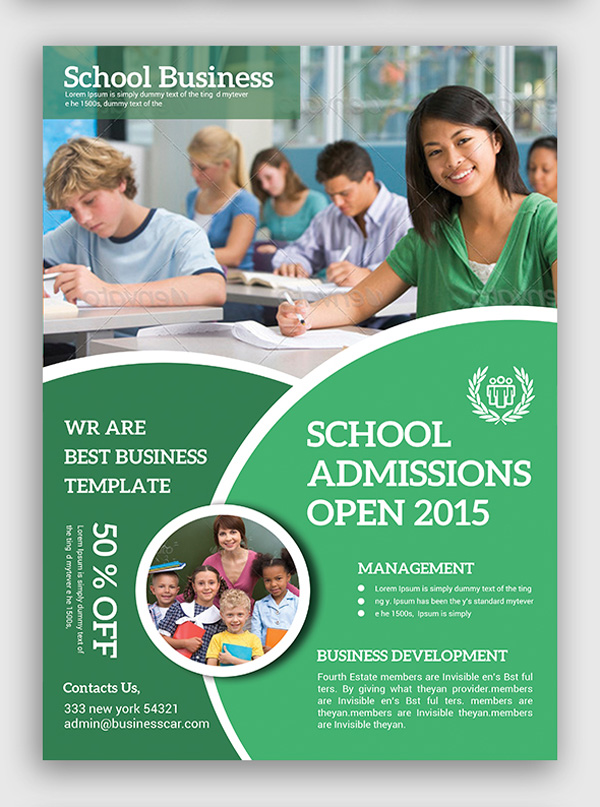The image depicts a scanned front cover of a school pamphlet that serves as a template. At the top left, the text "School Business" is displayed in white on a green banner. Below this, there's a stock image of a classroom where students, including a girl in a green shirt smiling at the camera, are seated and appear to be engaged in writing, perhaps taking a test. 

On the left side of the image, a prominent text reads "We are the Best Business Template," followed beneath by an offer that reads "50% off" and the contact information: "Contact us: 333 New York, 54321, admin@businesscar.com."

On the right side, the section titled "School Admissions Open 2015" is highlighted. Beneath it is a heading "Management" followed by three nonsensical bullet points. Below these points, another section reads "Business Development," followed by business-related sample dummy text.

At the bottom center of the flyer, there's an illustration of an adult with four children, enclosed in a circle. The overall content comprises placeholder text and random characters, indicating the flyer is a template, not finalized content.